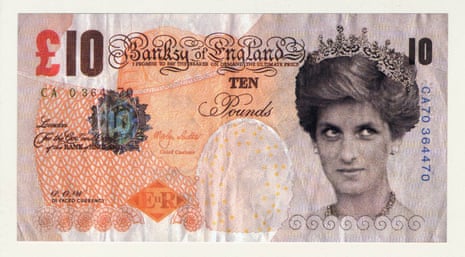This is an image of a 10 Pound currency note, featuring various hues of light pink, orange, gray, and white in the background. The note is presented in a landscape layout with a white border framing it. Prominently on the right side is a black-and-white portrait of Princess Diana, wearing a crown and a necklace, her image cut off at the chest and looking to the right. The upper left corner displays the pound symbol (£) in red with the number 10 in black. The same number 10 also appears in the upper right corner. Centrally, the text reads "Banksy of England" in black, with "10 Pounds" written directly below it. A blue serial number, CA70364470, runs vertically along the right-hand side. Additional features of the note include a blue seal and an orange seal on the left side, cursive black and orange text, various hollow marks, and yellow dots scattered in one area. The left side also contains a greenish-colored serial number and some signatures.